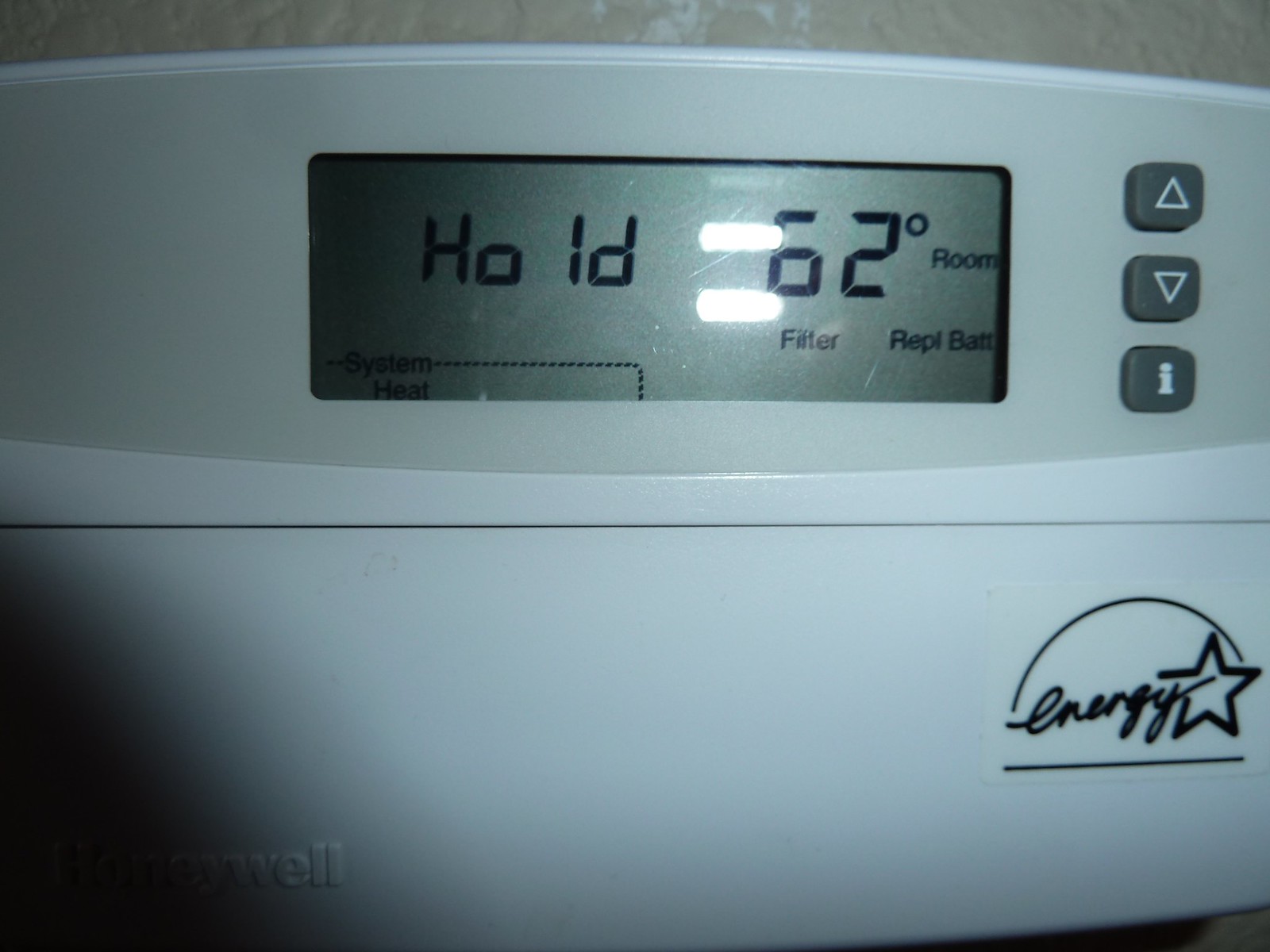This is a high-resolution color photograph depicting an in-home thermostat with a sleek design. Central to the image is a light gray screen that displays essential information. On the left side of the screen, the word "HOLD" is visible, albeit with a space separating the "HO" and "LD." To the right of this, the current room temperature is prominently displayed as "62 degrees." Below this, smaller text indicates statuses such as "filter," "rep," and "battery."

Adjacent to the screen on the right side, there are three rectangular buttons arranged vertically. The top button features an upward-pointing white triangle, the middle button has a downward-pointing white triangle, and the bottom button is labeled with a white letter "I," likely signifying an information function. All buttons share a grayish hue that contrasts slightly with the white symbols.

In the bottom right corner of the thermostat, an "Energy Star" label is printed in black ink. This label consists of the word "energy" accompanied by a star icon, all enclosed within a half-dome, semi-circular shape, indicating the energy efficiency certification of the device. The clean and organized layout of the thermostat, combined with the clear display and practical button arrangement, underscores its user-friendly interface and efficient functionality.